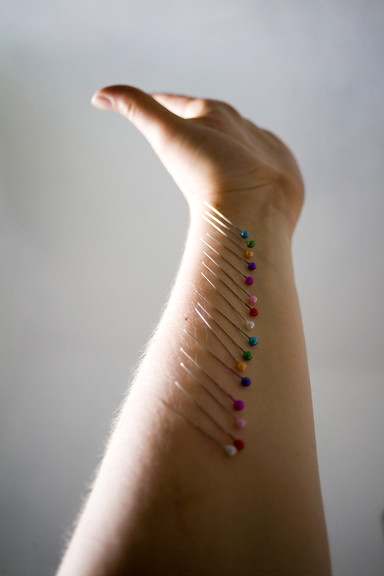This photograph features a person's right forearm extending upward against a medium gray background with a slight smoke-like gradient typical of professional photography. The individual's skin is a pinkish-white tone with faint pale body hair visible. The arm, possibly appearing double-jointed due to the hand's backward bend, is adorned with approximately twenty dressmaker pins. These pins, thin and sharp, are meticulously attached to the skin, running in a single line from the elbow to the wrist. Each pin boasts a colorful ball head, showcasing a variety of hues including red, blue, yellow, green, orange, white, and pink, making a striking and somewhat surreal visual impact.